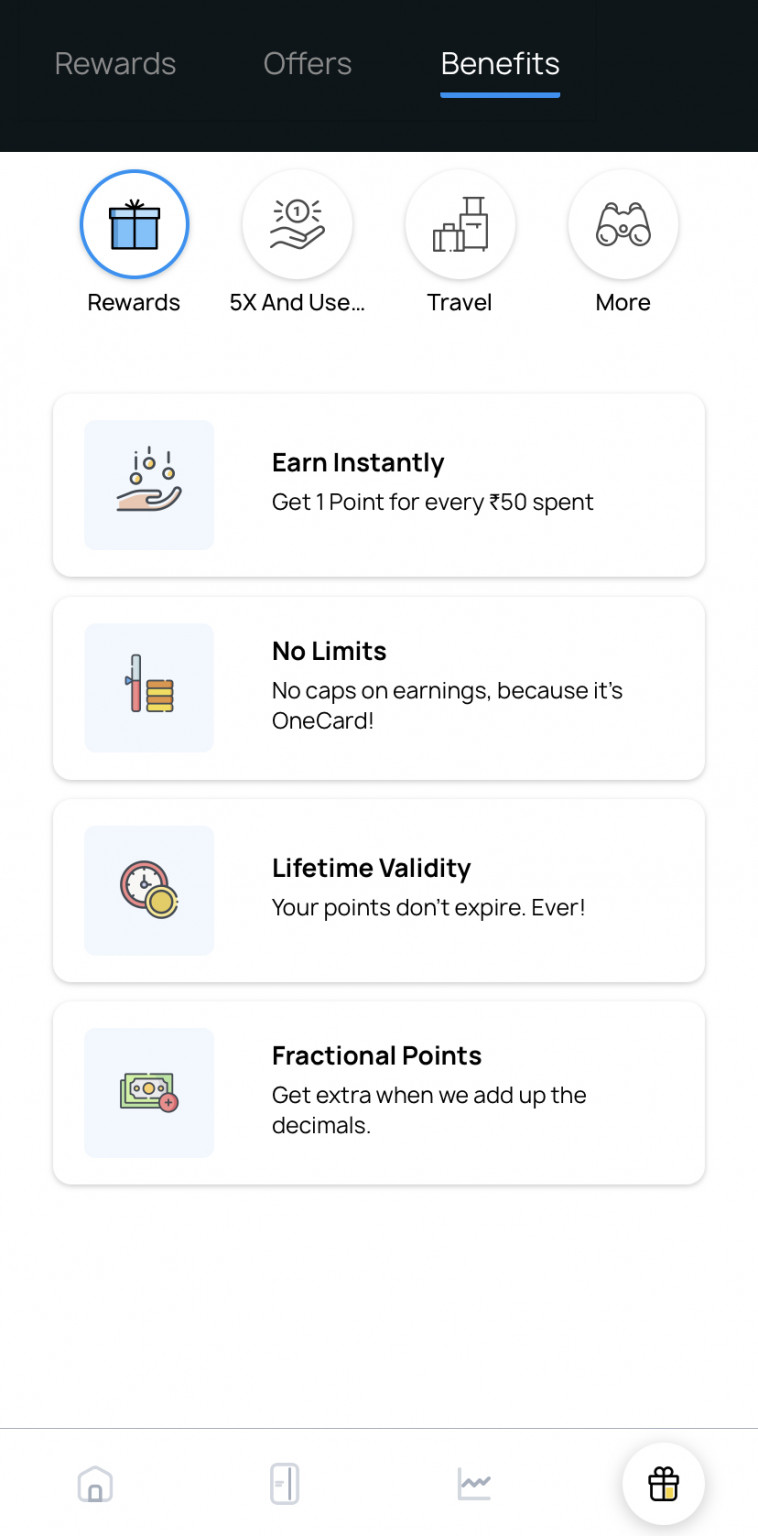Screenshot of a mobile app displaying the "Benefits" tab of a rewards program. The interface features three main tabs at the top: "Rewards," "Offers," and "Benefits," with the "Benefits" tab currently selected. Lower on the screen, there are different sections with labels such as "5X Rewards" and "Travel More." Several clickable links are visible, including "Earn Instantly," "No Limits," and "Lifetime Validity," alongside detailed descriptions such as "Fractional Points - Get extra when we add up the decimals." At the bottom, there are various navigation icons, including a home button and one resembling a present, likely indicating a rewards section. A unit of currency is displayed, though it is not in US dollars. The app appears to be associated with a rewards or loyalty program, potentially linked to a credit card, airline, or other service offering several ways to earn and use points.